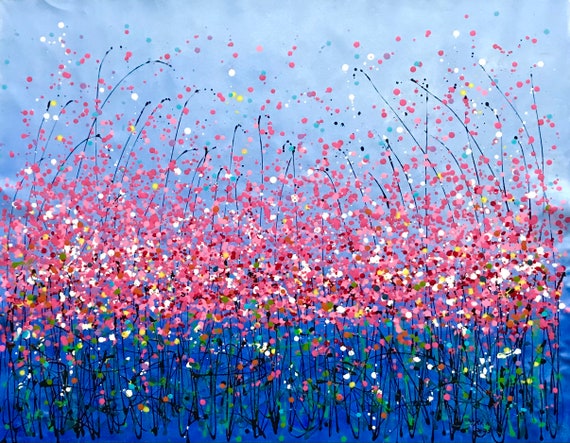This image depicts an intricate and vibrant abstract painting, strongly reminiscent of a Pollock-style artwork. The base of the square canvas is predominantly composed of royal blue paint, overlaid with vertical black lines stretching from the bottom towards the halfway point of the image. Scattered across this blue foundation are numerous specks and streaks of pink paint, which dominate the composition and evoke the playful and festive feeling of tiny pink flowers in a field.

Intermixed with the primary pink dots, there are also splashes of red, yellow, and green paint, adding complexity and depth to the picture without overshadowing the pink prominence. Above this base layer, the painting transitions into a depiction of a light blue sky, punctuated with various shades of blue and gray, mimicking the hues of a cloudy day. This sky section lacks distinct cloud forms, enhancing the abstract nature of the scene.

The combination of colorful specks and intricate lines result in a richly detailed image that marries the abstract with the impressionistic, inviting viewers to immerse themselves in a sea of vibrant, almost floral, celebration against a serene sky backdrop.